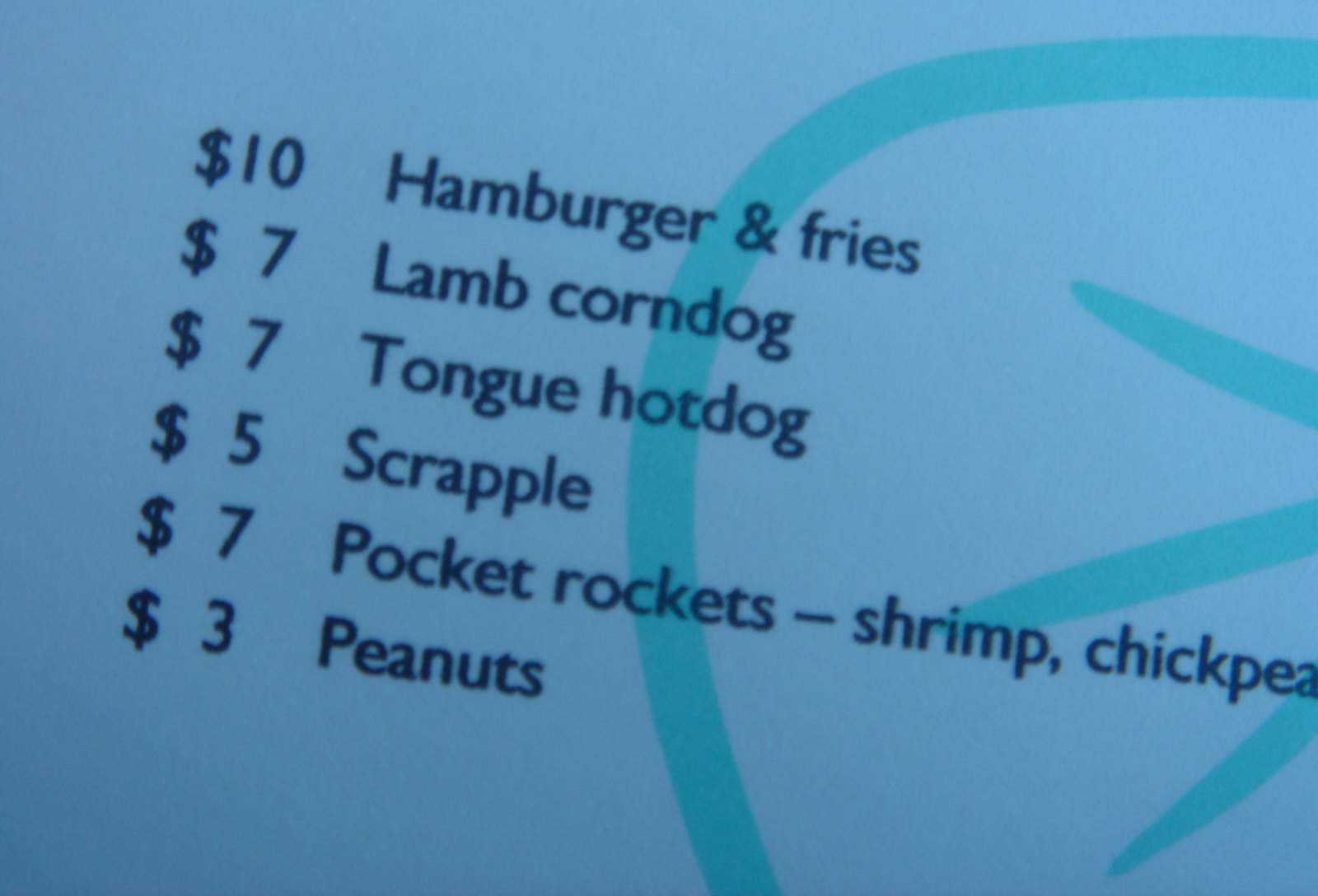This is a color photograph of a slightly tilted menu, with the text angled diagonally towards the bottom right. The menu is set against a white or light gray background, listing the items and their prices. The offerings include:

- Hamburger and Fries: $10
- Lamb Corn Dog: $7
- Tongue Hot Dog: $7
- Scrapple: $5
- Pocket Rockets (with Dash, Shrimp, Tom, and Chipotles): $7
- Peanuts: $3

On the right side of the menu, there is an outline of a green tomato.